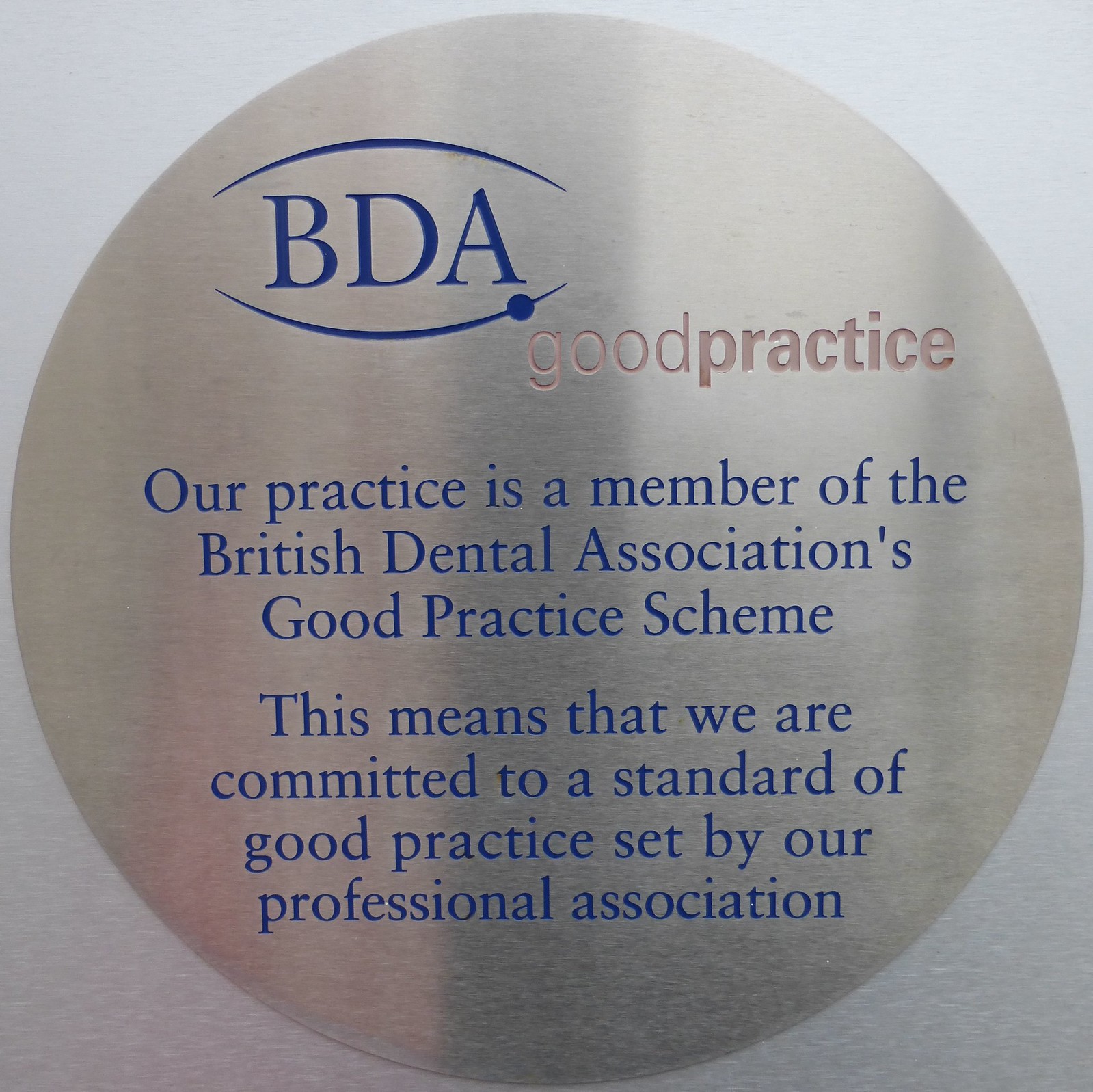The image depicts a close-up view of a round, metallic plaque, likely positioned against a white background. The plaque has a reflective surface with a gradient that transitions from a lighter greyish-blue at the top to a darker shade towards the bottom. Prominently engraved at the top are the initials "BDA," accompanied by a blue half-circle above and another below, with a blue dot beneath the bottom half-circle at the last bar of the 'A'. Immediately below, the words "good practice" are engraved, followed by the blue text: "Our practice is a member of the British Dental Association's Good Practice Scheme. This means that we are committed to a standard of good practice set by our professional association." The consistent theme and detailed craftsmanship suggest that this plaque is intended to reassure patients in a dental office of the practice's commitment to high standards as set by the British Dental Association.